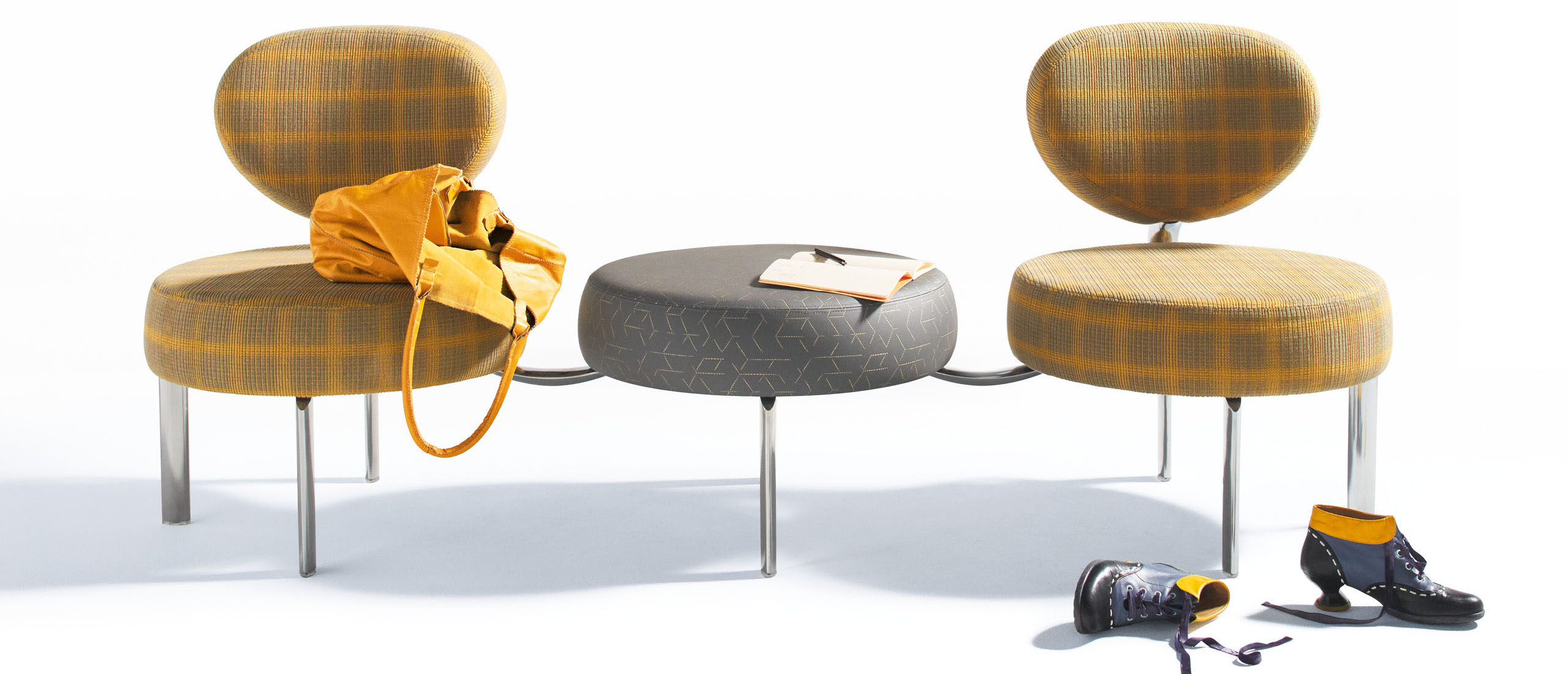This photograph features a unique seating arrangement against a white background. The image showcases three interconnected seats, each with metal legs and a curved metal rod linking them. The seating spots are all circular, with the outer two featuring backrests, while the middle one does not. The outer chairs are upholstered in a yellow and blue check pattern, whereas the central seat is entirely gray with a subtle line design. 

On the left chair, a yellow handbag rests with its handle slightly over the edge. The central seat holds an open notebook with a black pen placed on top. The right chair leads your eye to the floor, where a pair of distinctive high-heeled shoes in black, gray, and yellow tones are situated—one standing upright, the other toppled sideways. Shadows cast below suggest the arrangement is grounded. This composition juxtaposes everyday objects, bringing attention to their placement and design within the minimalist setting.